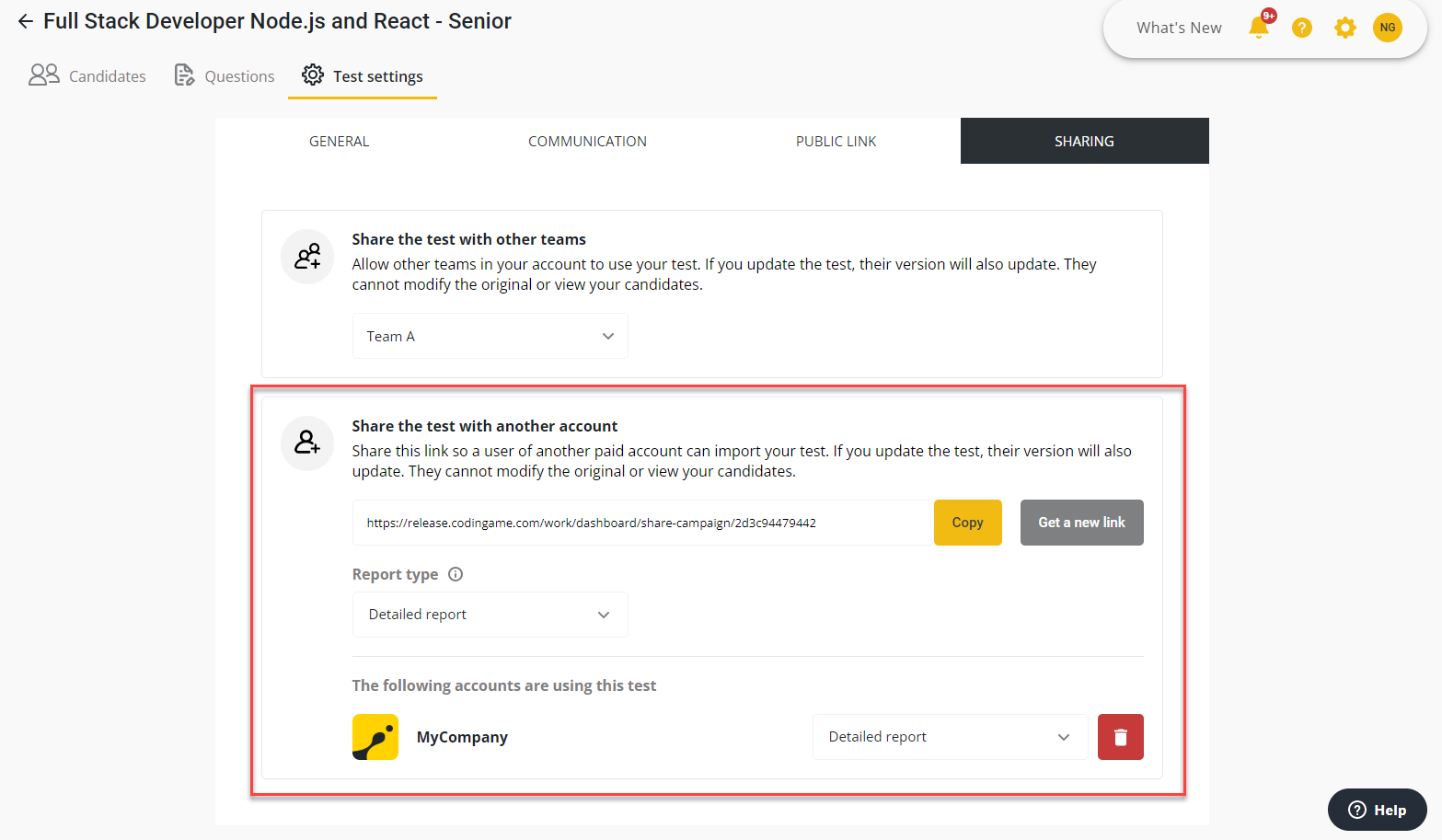The image is a screenshot taken from the desktop computer screen, showcasing an application interface likely used for managing recruitment tests. In the upper-left corner in black text, the title "Full Stack Developer Node.js and React - Senior" is displayed, indicating the focus of the interface. Below this title, there are three navigational options: "Candidates," "Questions," and "Test Settings," with "Test Settings" currently underlined, indicating it is the selected option.

The central area of the interface consists of a white rectangular window set against an off-white background. This window features four tabs at the top: "General," "Communication," "Public Link," and "Sharing," with the "Sharing" tab highlighted by a black rectangle, showing it is the active tab.

Within the "Sharing" tab, the interface is marked by a red-outlined rectangular section, which contains text and two buttons. A yellow button with black text reads "Copy," likely used to copy a link or information. Positioned next to this is a gray button with white text, though the specific text on this button is not clearly described.

The image provides a detailed view of an application designed to simplify and manage the different aspects of hiring a senior Full Stack Developer proficient in Node.js and React.